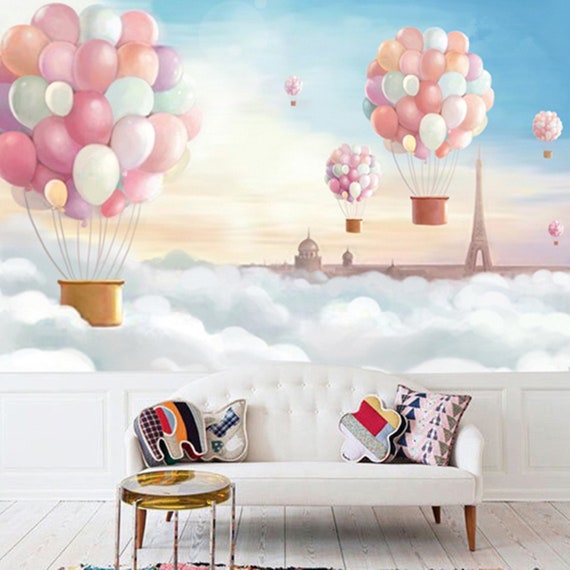The image appears computer-generated and depicts a whimsical living room with a light wood floor and white couch accented with various patterned pillows, including ones shaped like an elephant, butterfly, flower, and a plain square. In front of the couch, there's a small, round gold table. The lower half of the wall behind the couch is adorned with white wood block paneling, transitioning to a mural above. This mural presents a fantastical scene of pastel hot air balloons clustered together to form larger hot air balloons, floating against a backdrop of blue skies filled with fluffy clouds. Below the balloons, the Eiffel Tower and other monumental buildings suggest a Parisian setting. The room is brightly lit, conveying a sense of early daytime. A resin table and a furry rug complete the cozy and imaginative decor.